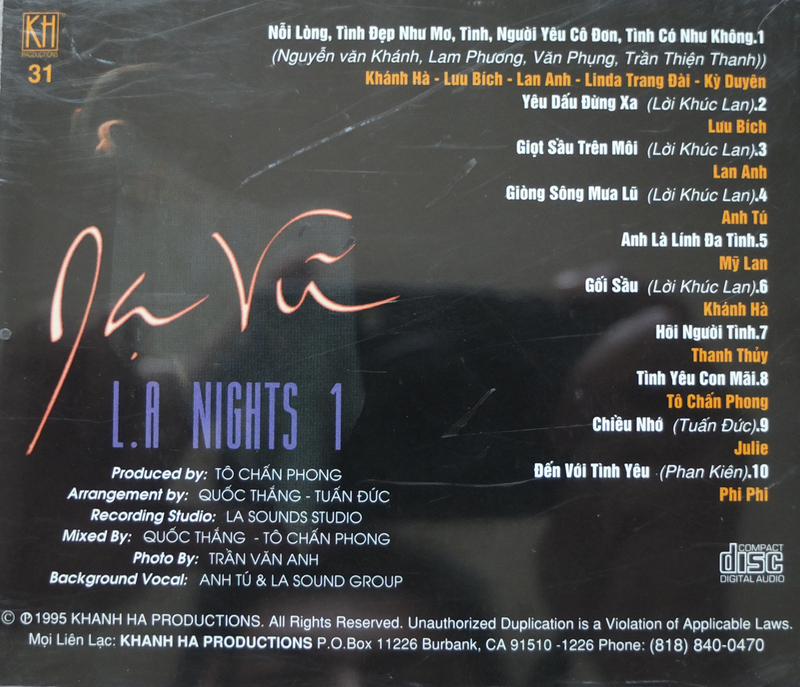This promotional advertisement features an album cover for the compact disc (CD) titled "LA Nights 1," produced by Conha Productions in 1995. The black background showcases vibrant text in white, orange, blue, and red. Positioned centrally, the CD cover prominently displays the "compact disc digital audio" symbol and lists the album's 10 Vietnamese song titles on the right side. The left side includes production details and credits, highlighting that the album artist is Jabu. Produced in Burbank, California, the production company’s details are listed, including their PO Box address (PO Box 11226, Burbank, CA 91510-1226) and phone number (818-840-0470).